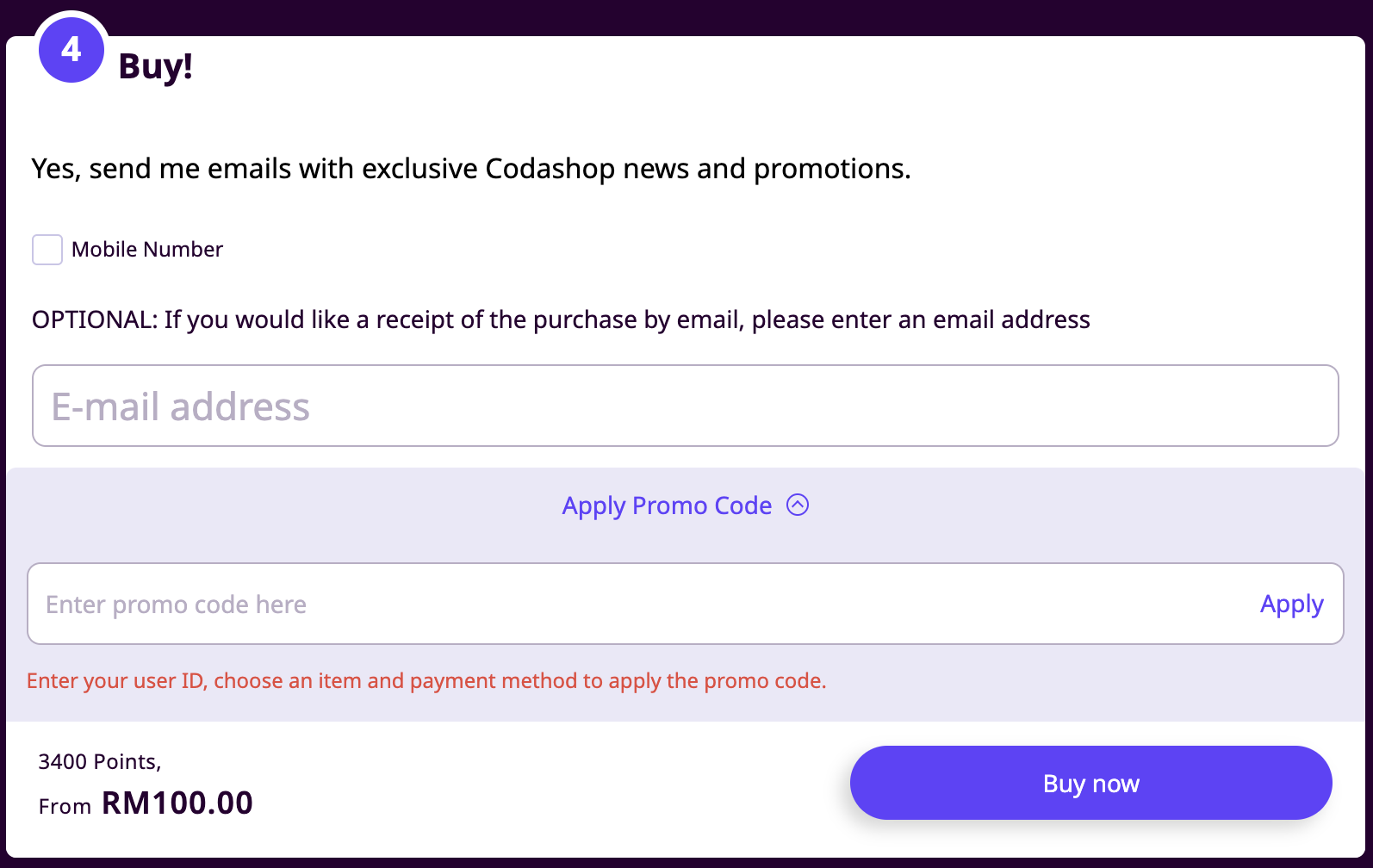This slightly rectangular image, with its dimensions, features a predominantly black background on the top, sides, and bottom edges. At the top left corner, a purple circle encloses a white numeral "4." To the right of this circle, the word "Buy" appears in black text. Beneath this, the phrase "Yes, send me emails with exclusive Kata shop news and promotions" is displayed. Below this sentence, there is a white checkbox labeled "Mobile number" to its right.

Further down, the image communicates in smaller text that providing an email address is optional and suggests entering an email address if you wish to receive a receipt of your purchase by email. A large input field underneath this prompt is designated for entering your email, and the placeholder text within this field reads "Email address."

At the center, the phrase "Apply promo code" is presented in purple letters on a slightly lighter purple background. Directly below, a white input box is provided for entering the promo code, with the placeholder text "Enter promo code here." To the right of this box, the word "Apply" appears in purple letters. Below this input area, red text instructs: "Enter your user ID, choose an item, and payment method to apply the promo code."

Toward the bottom left of the image, the text "3,400 points from RM 100.00" is written in dark purple letters. Finally, at the bottom right, a prominent purple button labeled "Buy Now" in white letters invites users to complete their purchase.